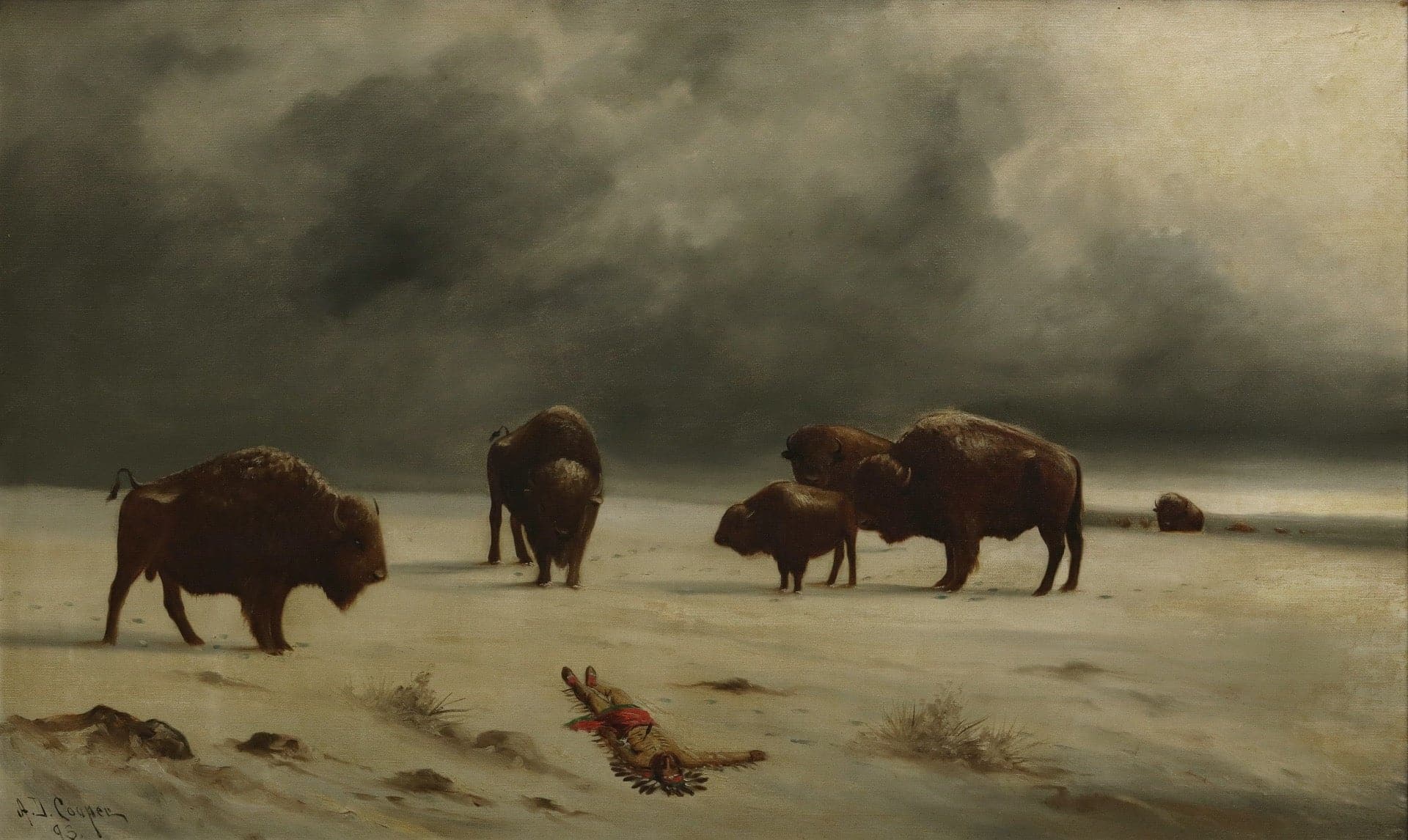The image depicts a dramatic and ominous outdoor scene, possibly a painting, capturing a moment reminiscent of the American West during its settlement period. The sky dominates the backdrop with thunderclouds swirling in shades of gray, black, and white, gradually blending into lighter hues of cream, yellow, and tan on the right side. Below this tumultuous sky, a herd of five buffalo, including one calf, stands prominently from left to right across the middle of the image. At the center of their attention is a Native American man lying flat on the sandy or stony ground. He wears a traditional headdress and has a bright red cloth covering his waist and groin area. His right arm extends outward at shoulder level, while his left arm lies by his side. The scene evokes a sense of mystery and foreboding, with more buffalo visible in the distance, approaching over a small hill, under the threatening sky.